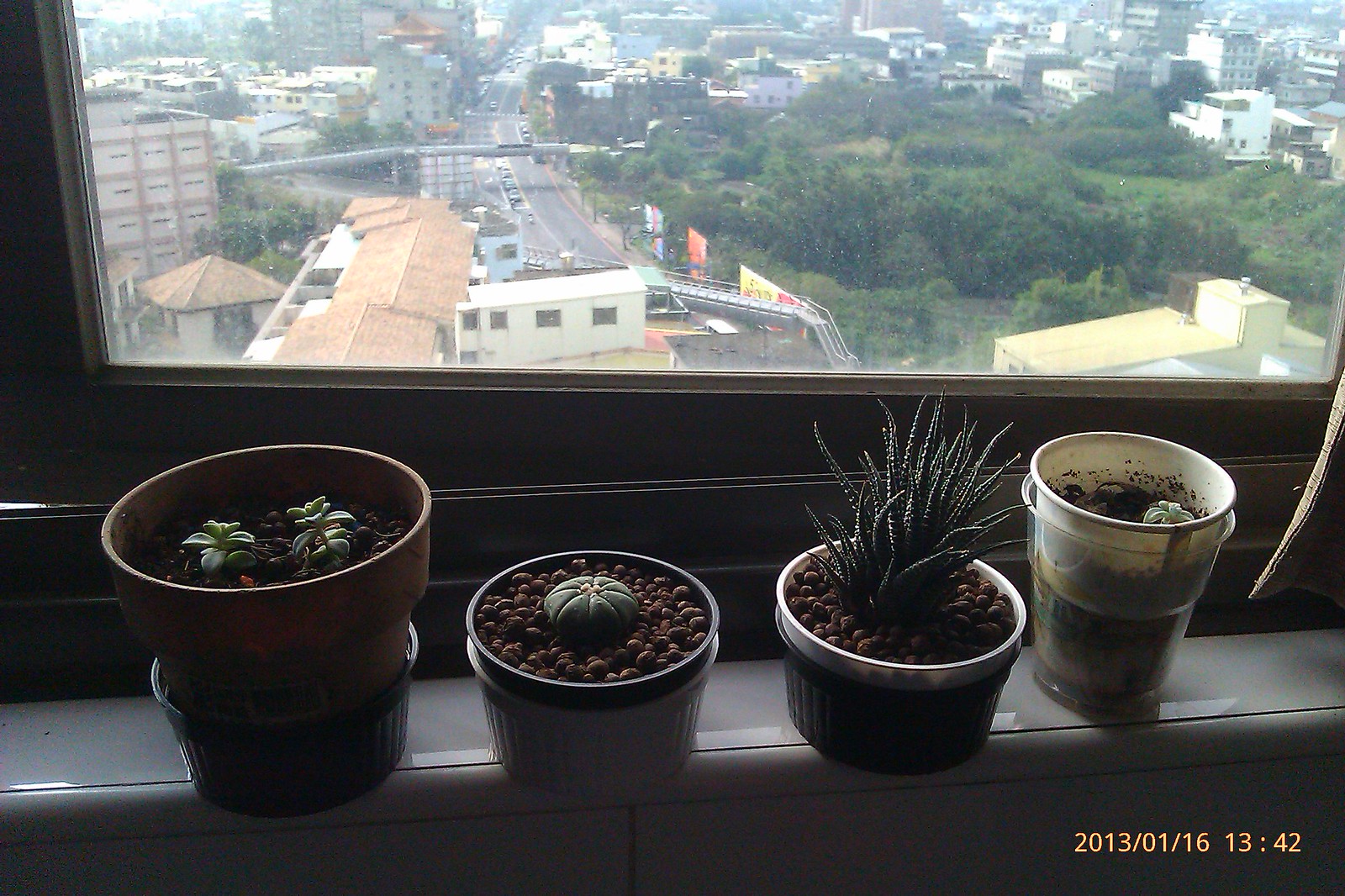The photograph captures a windowsill inside an apartment, overlooking an urban landscape. Four distinct plants in ceramic pots are lined up on the sill, with a dark gray window frame and sill. On the far left, a brown pot contains small sproutlings with pebbles on the soil. Next, a white pot holds a small green bulb, surrounded by stones resembling coffee pods. The third pot, black in color, has multiple green tendrils suggesting it might be a type of succulent or snake plant. On the far right, a white plastic container with a small leaf is placed inside a clear plastic cup. Above the windowsill, a large window offers a view of a cityscape with residential buildings, green parks, a main highway, and pedestrian bridges. The bottom right corner of the image is timestamped "2013-01-16, 13:42".